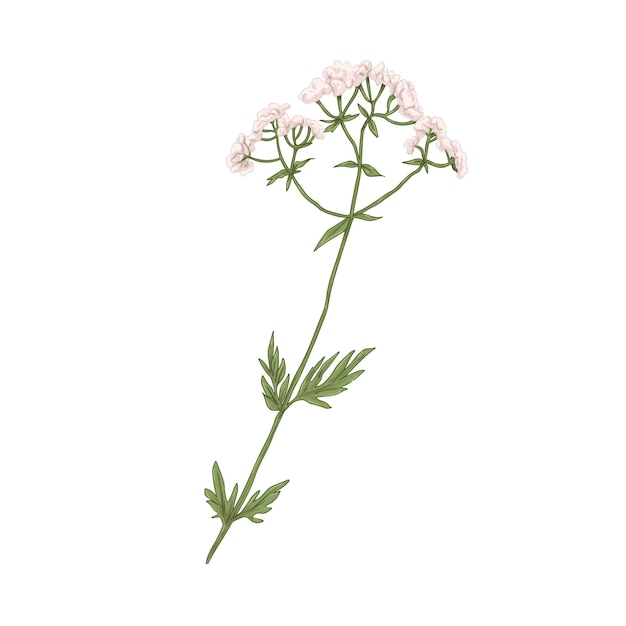The image is a simple yet detailed color pen and ink drawing of a flowering plant against a completely white background, giving it a slight 3D effect. The plant features a green stem starting from the lower left and extending to the upper right. Midway up the stem, there are small leaves arranged in sets, resembling a V-shape, with additional similar leaves spaced at thirds and halfway points. At the top of the plant, the main stem splits into three branches—one to the left, one to the right, and one continuing upward. These branches further divide into smaller sub-branches, each adorned with delicate pink flowers. The drawing’s meticulous details and the use of green and pink make it reminiscent of illustrations found in an herbarium or a scientific botanical book.